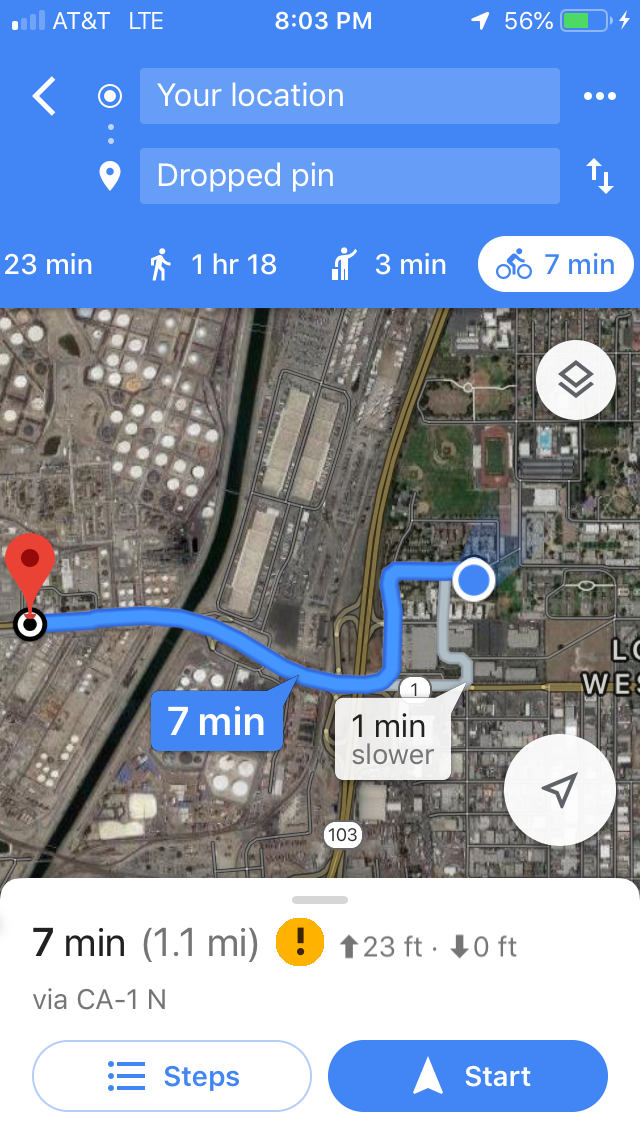The image depicts a detailed screenshot of Google Maps on a smartphone, displaying navigation options from the user's current location to a designated dropped pin. The chosen mode of transportation is biking, estimated to cover 1.1 miles in 7 minutes. Alternative routes are shown, with the primary path highlighted in blue and an alternate route, which is 1 minute slower, indicated in gray.

The status bar at the top of the screen shows that the device is connected to the AT&T network, albeit with just one bar of signal strength. The current time is prominently displayed as 8:03 PM, and the battery level is at 56%.

Additional details include the elevation change information, indicating an ascent of 23 feet and no significant descent. The screen layout suggests other travel times for comparison: a 7-minute walk and a 3-minute ride-hailing option, while walking the entire route would take approximately 1 hour and 18 minutes. The comprehensive visual provides a clear understanding of navigation options and real-time device status.